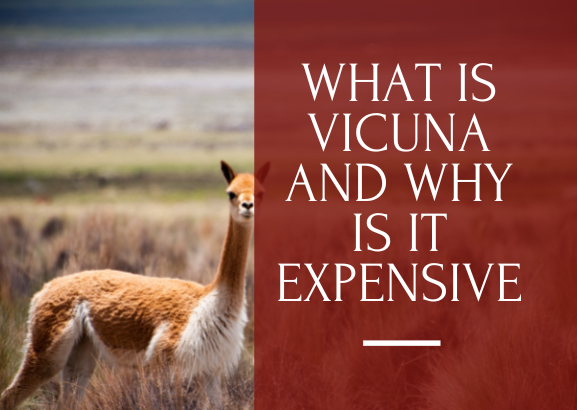The image depicts a llama standing in a grassy prairie setting, characterized by a distinct blend of brown and white fur. The llama features a long neck and a predominantly brown woolly back, with a white chest and subtle white markings around its mouth. The animal is gazing directly at the photographer, suggesting a moment of close attention. The photograph, taken outdoors under natural light, is horizontally oriented and rectangular in shape. On the right side of this image, there is a semi-transparent maroon banner with white text that reads, "What is Vicuna, and why is it expensive?" This text overlays the prairie scenery, adding an informative element to the picturesque scene.